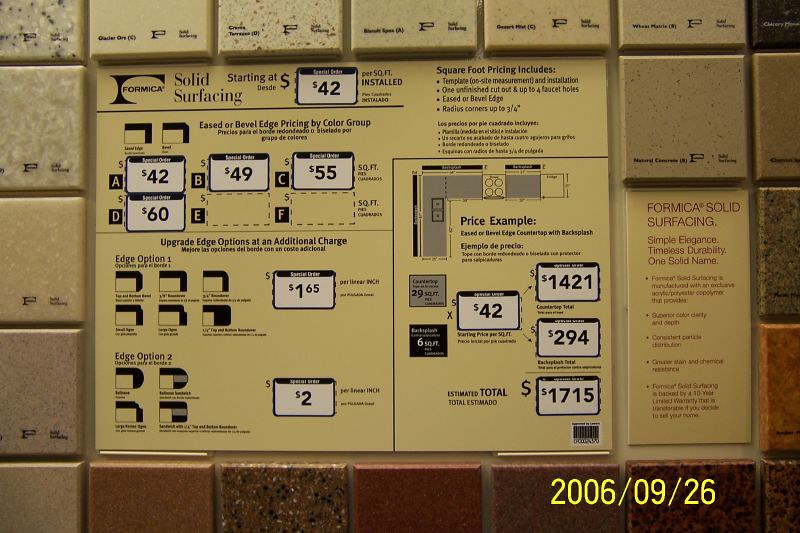This image portrays a beige wall adorned with intricate details including gray and red elements, possibly within a home improvement or material supply store. The focal point of the wall is a map-like layout advertising "Formica Solid Surfacing," with installation prices starting at $42 per square foot. The display includes various specifications and sample sizes of the material, suggesting product qualities and options available. The samples predominantly feature earthy tones, aligning with the rustic aesthetic highlighted in the other colors on the wall. This scene, likely captured on September 26, 2006, emphasizes Formica as an alternative to materials like granite, aimed at customers seeking laminate surfacing solutions for their homes.